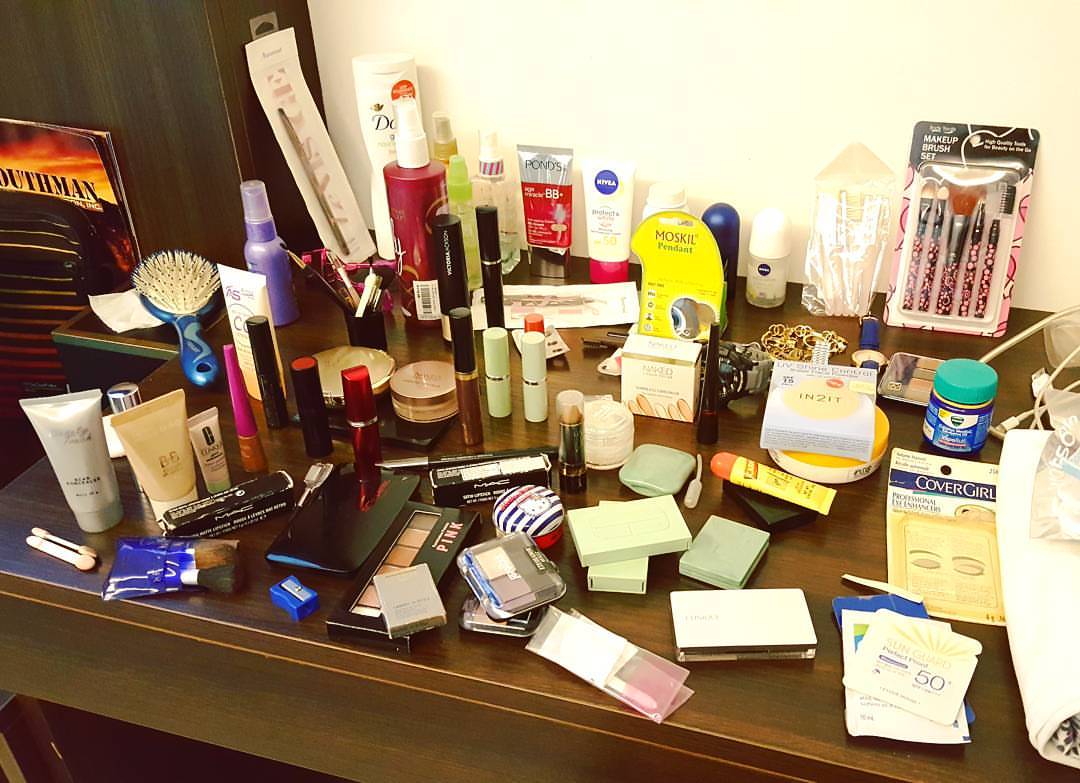A meticulously organized brown table is laden with an extensive array of beauty products. Dominating the scene, a variety of makeup brushes in different sizes and fullness are scattered across the surface, exuding an air of readiness for a thorough beauty regimen. Multiple lipsticks from MAC are prominently featured alongside disposable eyeshadow applicators, eyeshadows, false eyelashes, and both liquid and powder foundations. Complementing them are essential items such as deodorant, hairspray, Vicks, sunscreen, and an assortment of face creams. A handful of makeup tools, including hairbrushes, eye brushes, and a Carmex lip balm, add to the cluttered yet purposeful setup.

In addition, a sprinkling of jewelry is evident, with a gold necklace and a ring casually placed near the assortment. Next to them lies a small silver tray, perfect for storing earrings or rings. Charging cords snake through the beauty products, hinting at a multitasking space. Nivea lotion and Dove products further contribute to the mix, while three identical cases of beauty products add to the abundance. This image offers a fascinating glimpse into a beauty enthusiast’s well-stocked and varied collection.